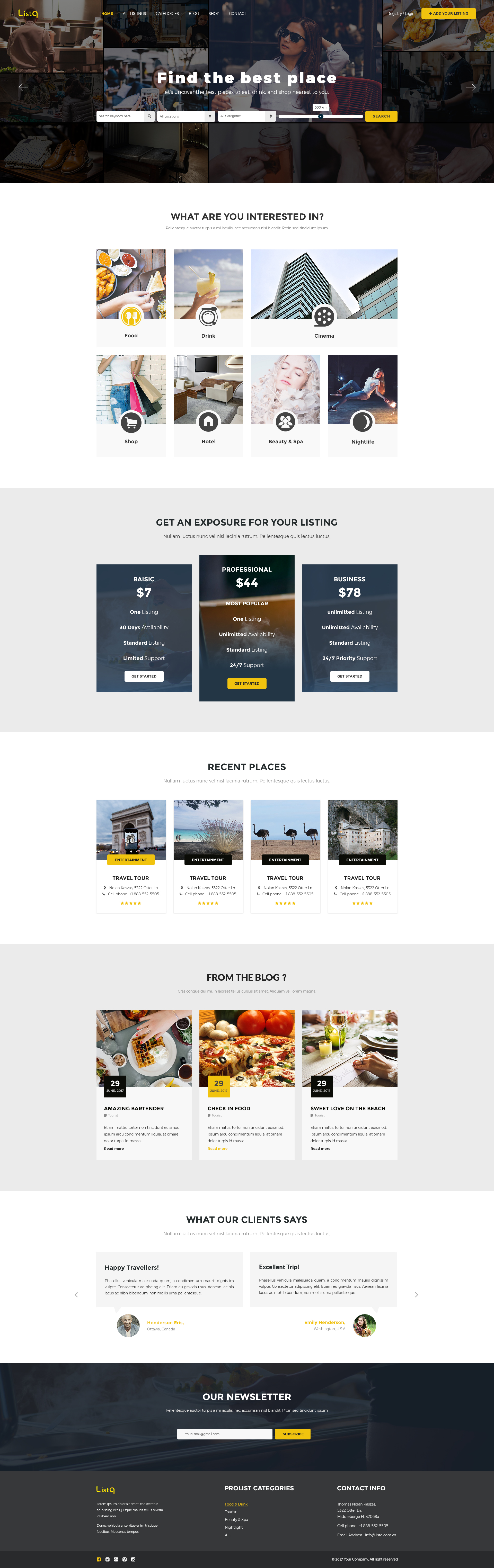In this image, we observe a user interface layout designed for a web or mobile application centered around finding and listing places of interest. 

At the very top left, there is a logo or name beginning with an "L," potentially "Lark," though the text appears quite small and difficult to read. 

In the top center, a prominent phrase in white text reads, "Find the best place." Directly below this, there are several input fields where users can enter search information.

Moving further down, the heading "What are you interested in?" is followed by a grid of seven selection boxes labeled with various categories: "Food," "Drinks," "Home," "Sleep," "Hotel," "Beauty & Spa," and "Dance."

Beneath these categories, another section is focusing on listing exposure, titled "Get an exposure for your listing." Three pricing options are presented here: the first box on the far left states "Basic for $7," the middle box offers "Professional for $44," and the third box on the right provides "Business for $78."

Below the pricing options, the section titled "Recent places" features four boxes with diverse images depicting archways, animals, and a beach scene, hinting at different locations or attractions.

Further down, there's another segment labeled "From the blog," highlighting three blog categories, each supplemented with appealing images of food.

Finally, at the bottom, there is a section named "What our clients say," which contains two review boxes showcasing client testimonials.